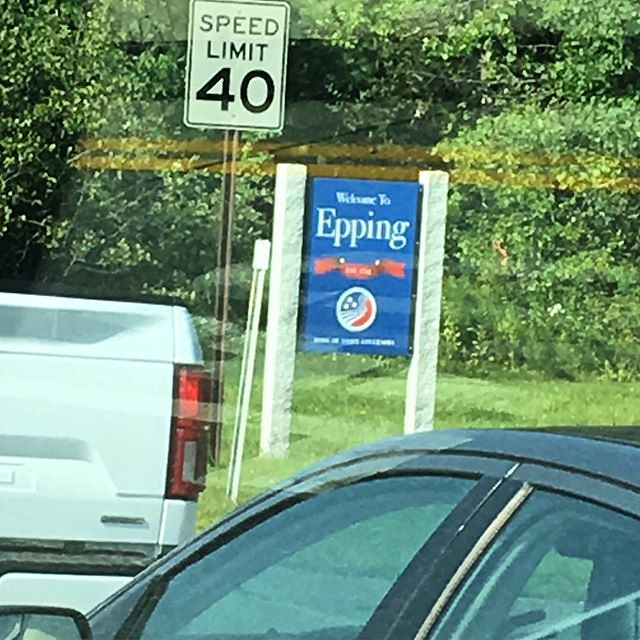The color photograph appears to be taken from inside a car, through a window, as a faint reflection spans across the image. The scene captures the side of a road on a bright, sunny day. Dominating the center of the image is a blue rectangular sign with white lettering that reads, "Welcome to Epping." Flanked by two white posts, the sign sits on a well-manicured green lawn, adorned with a red banner below the text and a white circle featuring a red, white, and blue emblem. Just in front of this welcome sign, a white metal pole holds a speed limit sign indicating "Speed Limit 40." To the left of the speed limit sign, the back of a white pickup truck with a visible red taillight is captured, while to the right, there's a dark-colored, likely black or gray, four-door sedan. Surrounding the welcoming sign and speed limit indicator is a backdrop of lush green shrubs and trees, emphasizing the bright and clear daylight of the scene.